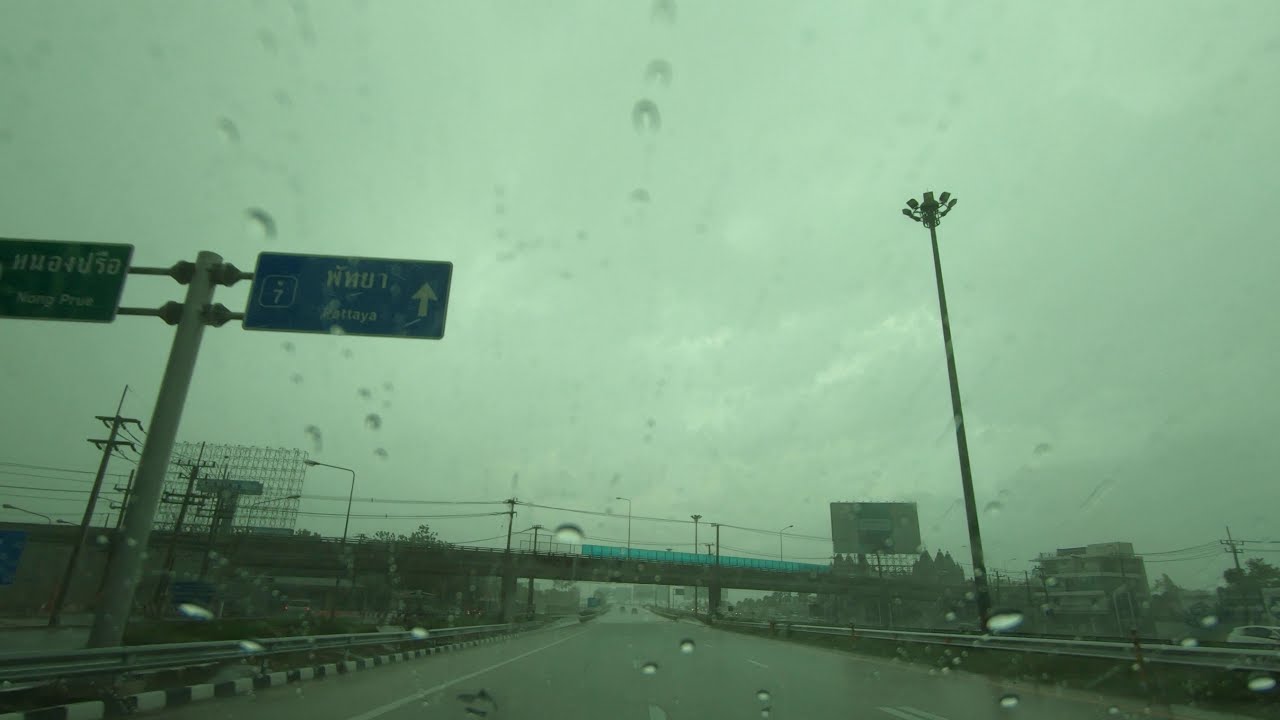A photograph taken from inside a moving car on a multi-lane highway captures a rainy, overcast day. Through the windshield, which is dotted with water droplets, the road stretches ahead with visible white dashed lines. Metal guardrails line both sides of the highway. On the right side, a tall lamppost rises above, and further afar, a multi-story building and a billboard are visible. To the left, a blue and white street sign with an arrow and a hefty steel structure can be seen. The car is approaching an overpass that spans the road, featuring green netting along its sides. The sky, occupying the upper two-thirds of the frame, is a stormy blend of gray and green hues, casting a dreary tint over the entire scene. In the background on the far left, an industrial area with telephone poles and large equipment is faintly visible, adding to the photo's overall somber and hazy ambiance.